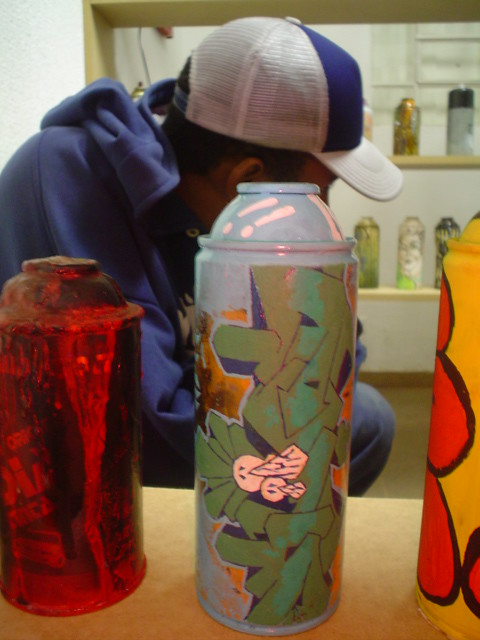This detailed photograph captures the scene of a young man, possibly a graffiti artist, seated behind a beige-colored surface. The man, whose face is turned away from the camera, has dark brown hair and is wearing a white and blue baseball cap with a royal blue front and a white visor. He is dressed in a blue hoodie, and blue jeans, further emphasizing his casual appearance. In the foreground on the light beige surface, there are three spray cans prominently displayed. 

The spray can on the left is a well-used red canister, its label obscured by layers of dried paint. In the middle, there is a light blue and green can, which features intricate graffiti designs. The can on the right, slightly out of frame, is primarily white with red accents and has a transparent dark red appearance. Each can shows signs of heavy usage, characteristic of a seasoned artist's tools. 

Behind the man, there is additional shelving populated with more spray cans and containers, showcasing a variety of colors like tan, white, pink, and yellowish tones. These shelves further hint at the setting being indoors, likely a workspace dedicated to the artist's craft. The detailed arrangement of the cans and the attire of the individual suggest a snapshot into the world of a passionate graffiti artist.